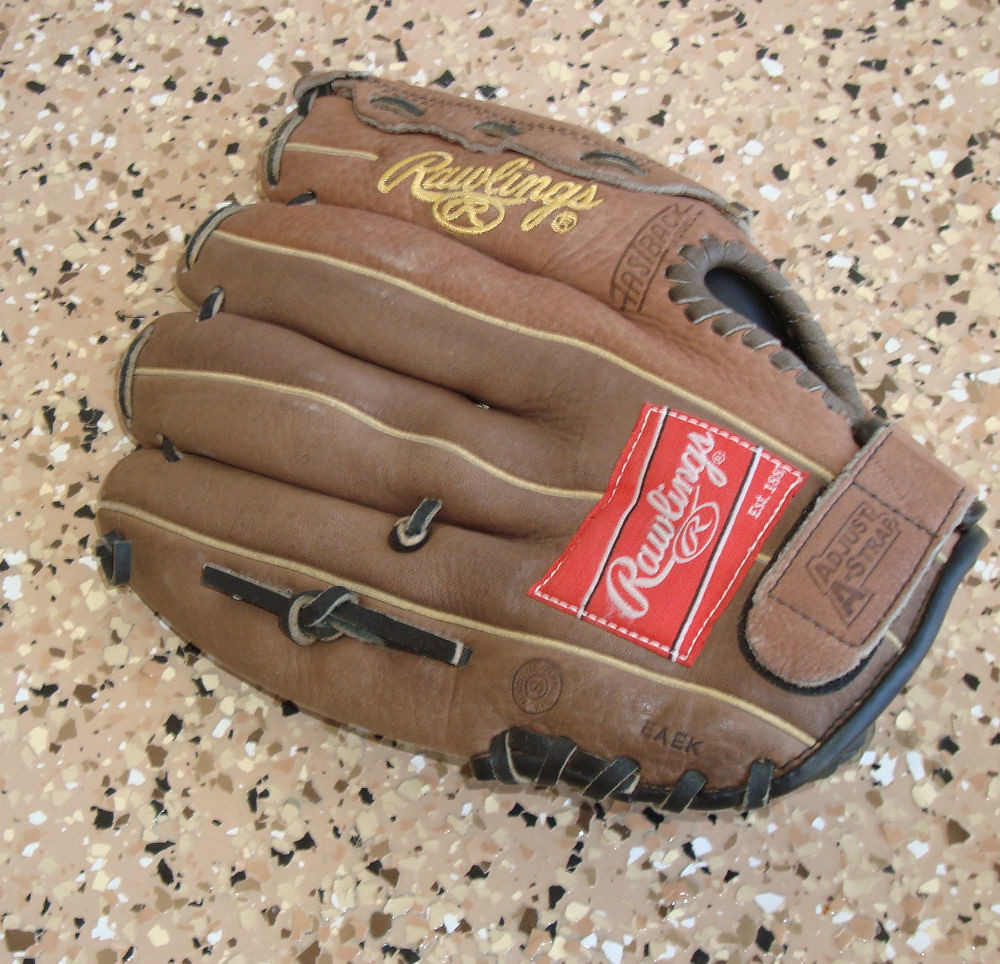The image showcases a medium brown leather Rawlings baseball mitt, prominently displaying the Rawlings logo with yellow print across the upper finger area, accompanied by a red label near the wrist that reads "Rawlings, Established 1857." The mitt is placed palm down on a kitchen countertop featuring a mottled pattern of beige, black, white, and dark brown speckles, harmoniously blending with the glove's color. The design includes detailed leather stitching and lacing around the edges, with a cocoa brown velcro strap at the wrist that reads "Adjust a Strap." The trimmings and some of the stitching are in darker brown or black, highlighting the craftsmanship of the glove. The glove is positioned slightly diagonally on the countertop, further drawing attention to its intricate details and high-quality leather material.